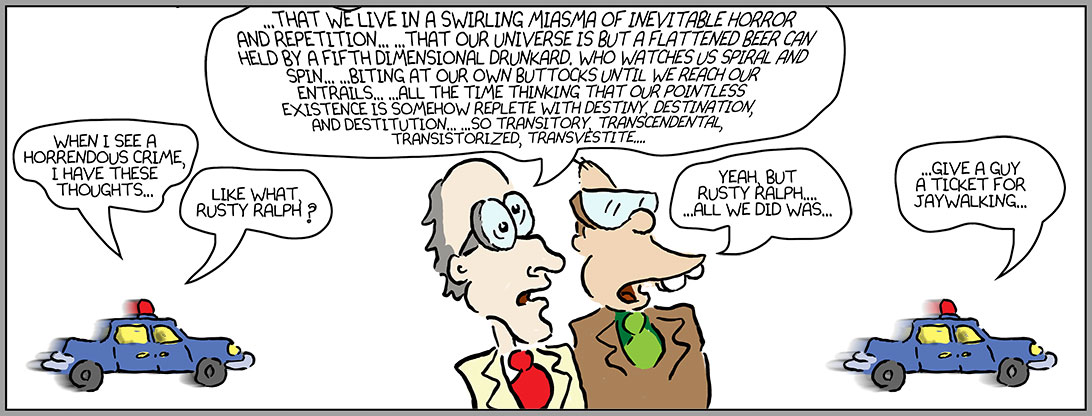The image depicts a detailed comic strip, set against a white background, featuring two cartoonish older men standing in the center, facing the viewer. Both men wear glasses and professional attire, with the man on the left in a cream suit and red tie and the man on the right in a brown suit and green tie. Flanking these characters on the left and right sides are blue police cars with red lights on top. The left police car has a speech bubble saying, "When I see a horrendous crime, I have these thoughts. Like what, Rusty Ralph?" The center of the comic showcases the two men, with the man in the cream suit delivering a lengthy, existential monologue: "That we live in a swirling miasma of inevitable horror and repetition, that our universe is but a flattened beer can held by a fifth-dimensional drunkard who watches us spiral and spin, biting at our own buttocks until we reach our entrails, all the time thinking that our pointless existence is somehow replete with destiny, destination, and destitution. So transitory, transcendental, transistorized, and transvestite." The other man responds, "Yeah, but Rusty Ralph, all we did was," at which point the police car on the right completes the thought with, "give a guy a ticket for jaywalking."